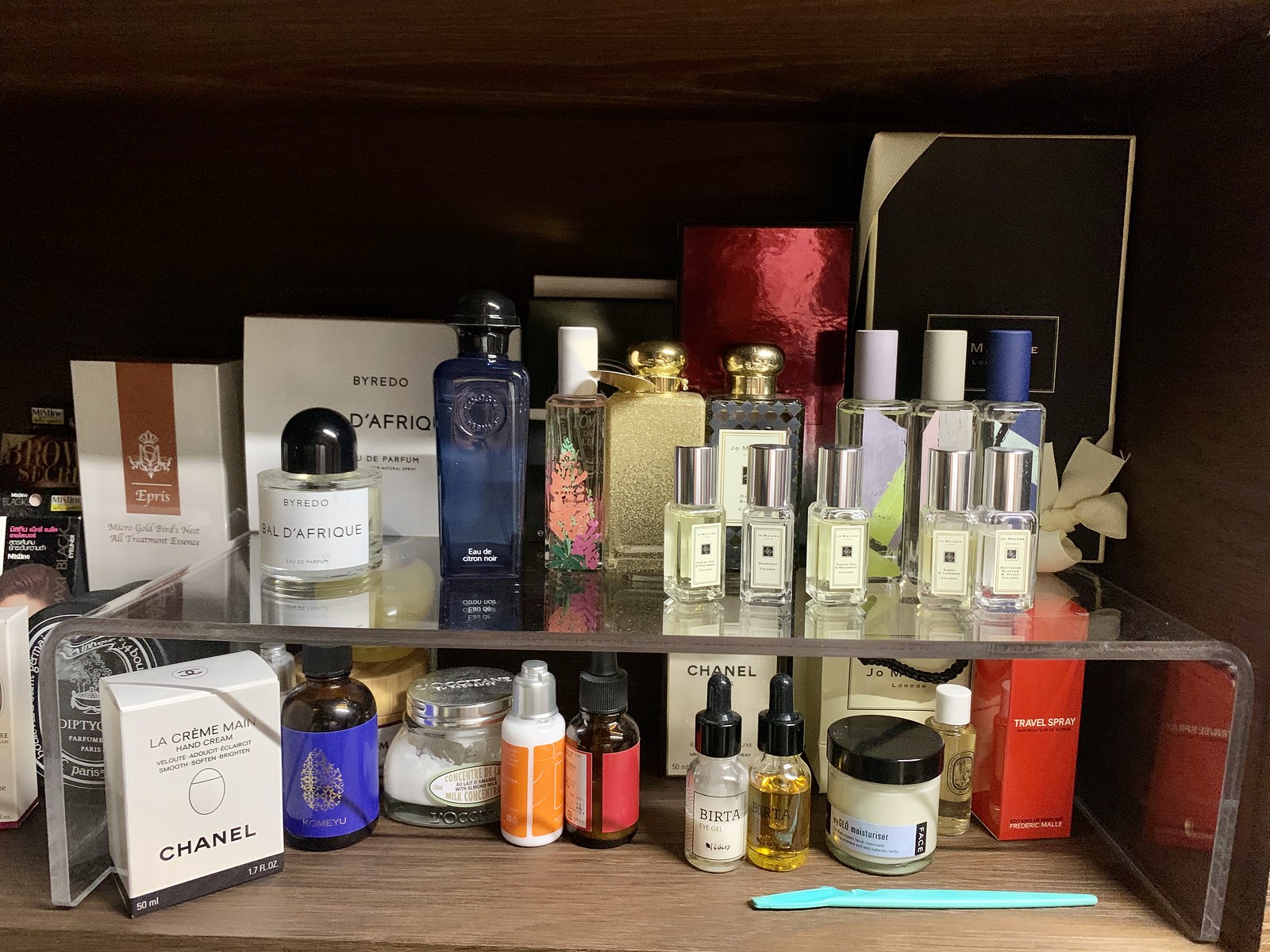This photo showcases an intricate display of fragrances and cosmetics, meticulously arranged on a beautifully crafted wooden surface that resembles a table or floor. The landscape-oriented image captures a display enclosed in a wooden frame, creating a boxed-in look with the sole opening facing the viewer.

The backdrop and sides are constructed from the same wood-like material, which extends up the right side, across the top, and partially along the left side before being cut off by the photo’s edge. At the back, a wooden cover completes the enclosure, adding to the framed aesthetic of the setup.

On a clear glass or plastic shelf within the display, two rows of assorted products are organized neatly. On the top right, several small bottles with silver tops are filled with a yellowish or greenish liquid. Behind them, equally sized bottles with blue, silver, and white caps feature clear bases, creating a harmonious pattern. A prominent black box is positioned in the back right corner, accompanied by a large red box to its left.

To the left on the top shelf, a blue perfume bottle stands out among the arrangement, next to a unique circular clear bottle capped with a semi-circle black top. Below, on the bottom layer of the shelf, an array of small bottles and miscellaneous items are scattered, including a notable white Chanel box. These items collectively exude an impression of a high-end fragrance and cosmetic collection, evoking sophistication and elegance.